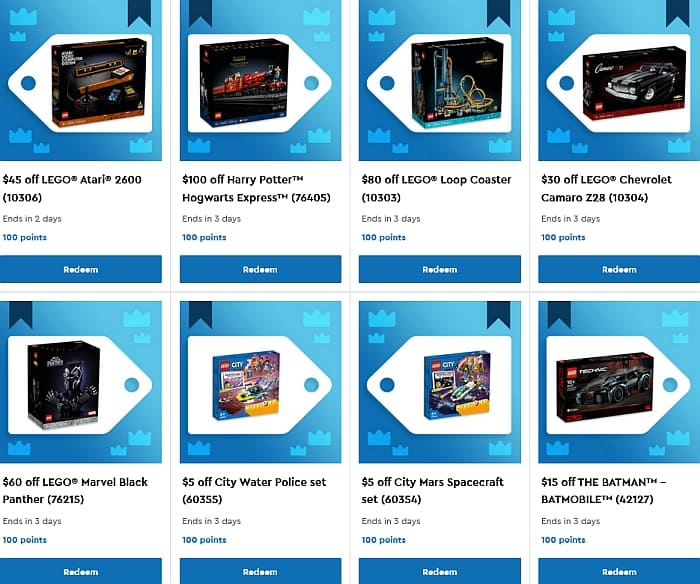This image features a visually appealing layout showcasing eight children's toy sets arranged in a grid of four columns and two rows. The toys are displayed within a blue box adorned with small crown graphics, giving a playful and royal touch. Each toy box appears identical in shape and size and includes a classic white price tag graphic, enhancing the aesthetic of a retail display.

The toys highlighted include: 
- Lego Loop Coaster
- Lego Chevrolet Camaro
- City Water Police Set
- Atari
- Harry Potter Hogwarts Express

These toys are themed around automobiles and racing sets, invoking a sense of adventure and speed. Each item is associated with a discount coupon, visibly marked with savings such as '$45 off' and clickable options to redeem these offers. The time sensitivity of the deals is indicated with "Ends in 3 days" or "Ends in 2 days." Each coupon is valued at 100 points, making the offers enticing for potential buyers.